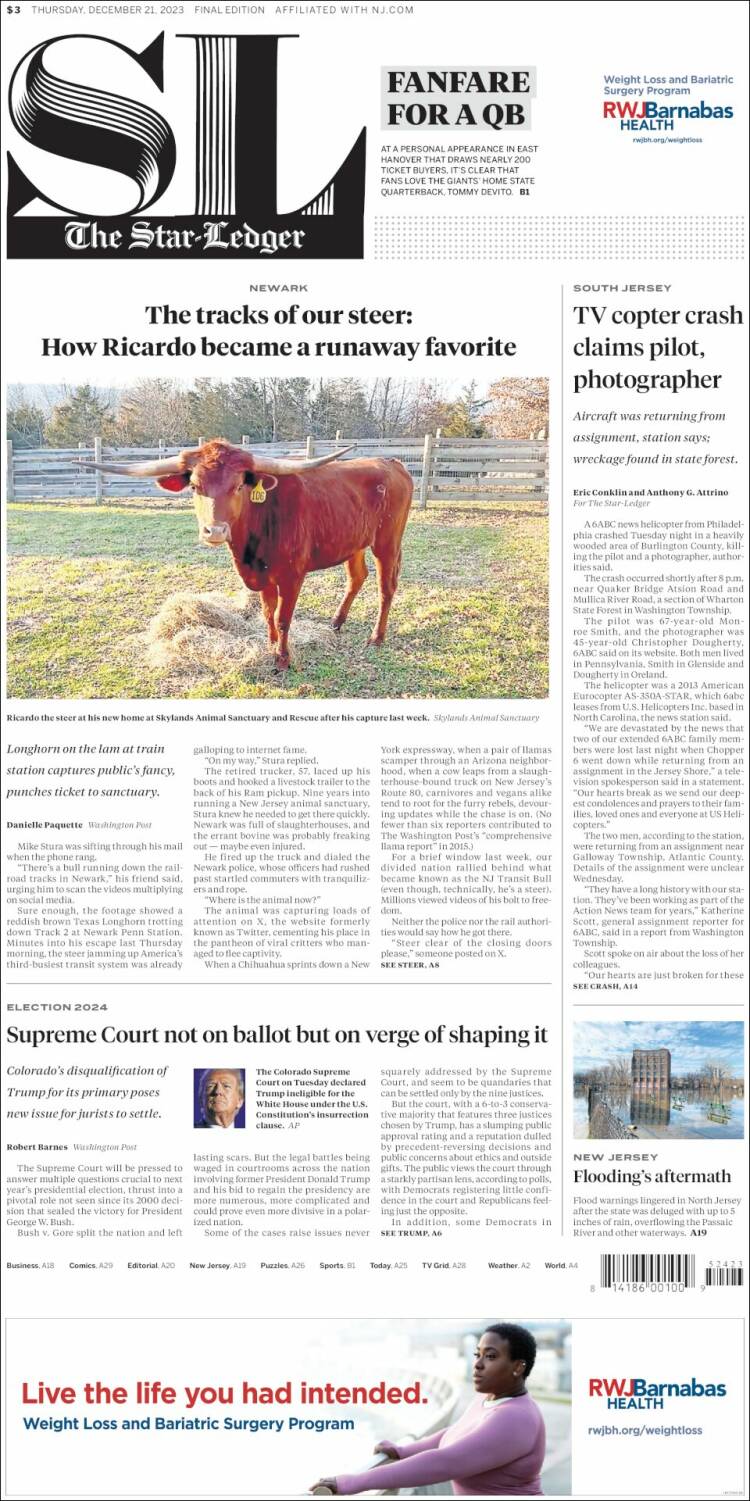This is a detailed screenshot of a newspaper, specifically "The Star-Ledger," easily identifiable by its black masthead at the top reading "SL The Star-Ledger." In the upper section, there's an advertisement for "Fan Pier of QB." Adjacent to it, on the right, there's a smaller ad promoting weight loss and bariatric surgery services by RWJ Barnabas Health.

The headline dominates the page with a large photograph of a cow or bull, complete with visible horns and a tag, standing in a field with a fence in the background. The caption reads, "The Tracks of Our Steer: How Ricardo Became a Runaway Favorite," introducing a prominent story.

Beneath this main article lies another story with a portrait of a person. The headline states, "Supreme Court Not on Ballot but on Verge of Shaping It." To its right, there's another significant story headlined, "TV Copter Crash Claims Pilot and Photographer."

Further down the page, there is a smaller feature labeled "New Jersey Flooding Aftermath," accompanied by an image depicting a flooded city.

At the bottom of the page, a large advertisement showcases a woman in a violet long-sleeved shirt. The advertisement promotes a weight loss and bariatric surgery program by RWJ Barnabas Health, with the encouraging tagline, "Live the Life You Had Intended."